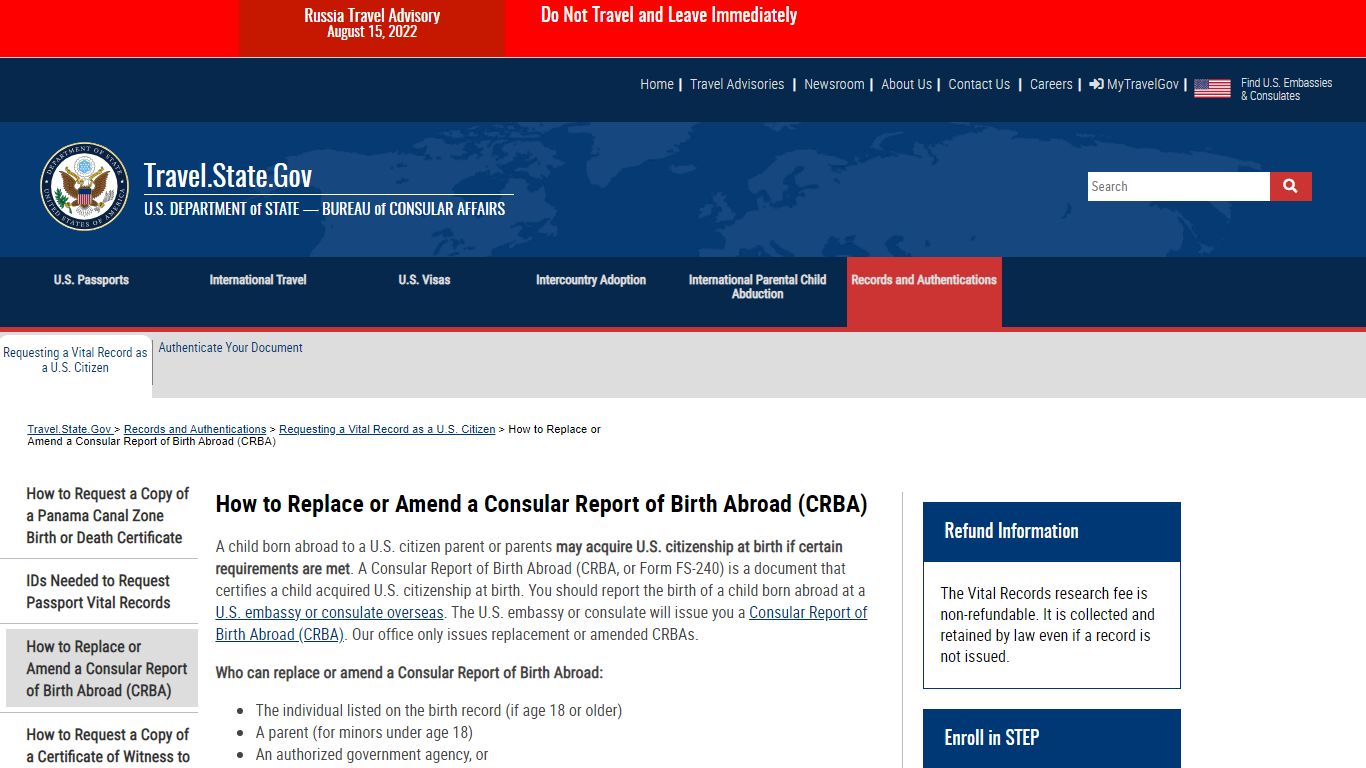The government website prominently displays a red banner at the top which reads, "Russia Travel Advisory - August 15, 2022: Do Not Travel and Leave Immediately." Directly beneath this, the website shifts to a blue header featuring several navigation tabs on the right-hand side: Home, Travel Advisory, Newsroom, U.S. Contact Us, Careers, and MyTravelGov.

An American flag is visible, followed by a link labeled "Find U.S. Embassies and Consulates." Below this, the emblem of the Department of State, United States of America, featuring an eagle, is prominently displayed. Next to the emblem, the text "Travel.State.Gov" appears in white, along with a logo indicating it is the "U.S. Department of State, Bureau of Consulate Affairs."

To the right of this, a white rectangular box with the label "Search" in gray is visible, adjacent to a red box containing a white magnifying glass icon for search functionality. 

Below these elements, several informational sections are listed: 

- How to request a copy of a Panama Canal Zone Birth or Death Certificate.
- IDs needed to request a passport or vital records.
- How to replace or amend a Consular Report of Birth Abroad.
- How to request a copy of Certificate of Witness to Marriage.

One detailed section explains the process of replacing or amending a Consular Report of Birth Abroad (CRBA), highlighting that a child born abroad to U.S. citizen parents may acquire citizenship at birth if certain requirements are met. The Consular Report of Birth Abroad is a document certifying this citizenship. Births should be reported at the U.S. Embassy or Consulate overseas, which will issue the CRBA. The website notes that the office only issues replacements and amendments to existing CRBAs.

Eligibility for replacing or amending a CRBA includes:
- An individual listed on the birth certificate, if aged 18 or older.
- A parent for minors under the age of 18.
- An authorized government agency.

This informational layout ensures that visitors can easily navigate and understand the essential travel advisories and procedures related to obtaining vital records while also making vital immigration and citizenship information accessible.